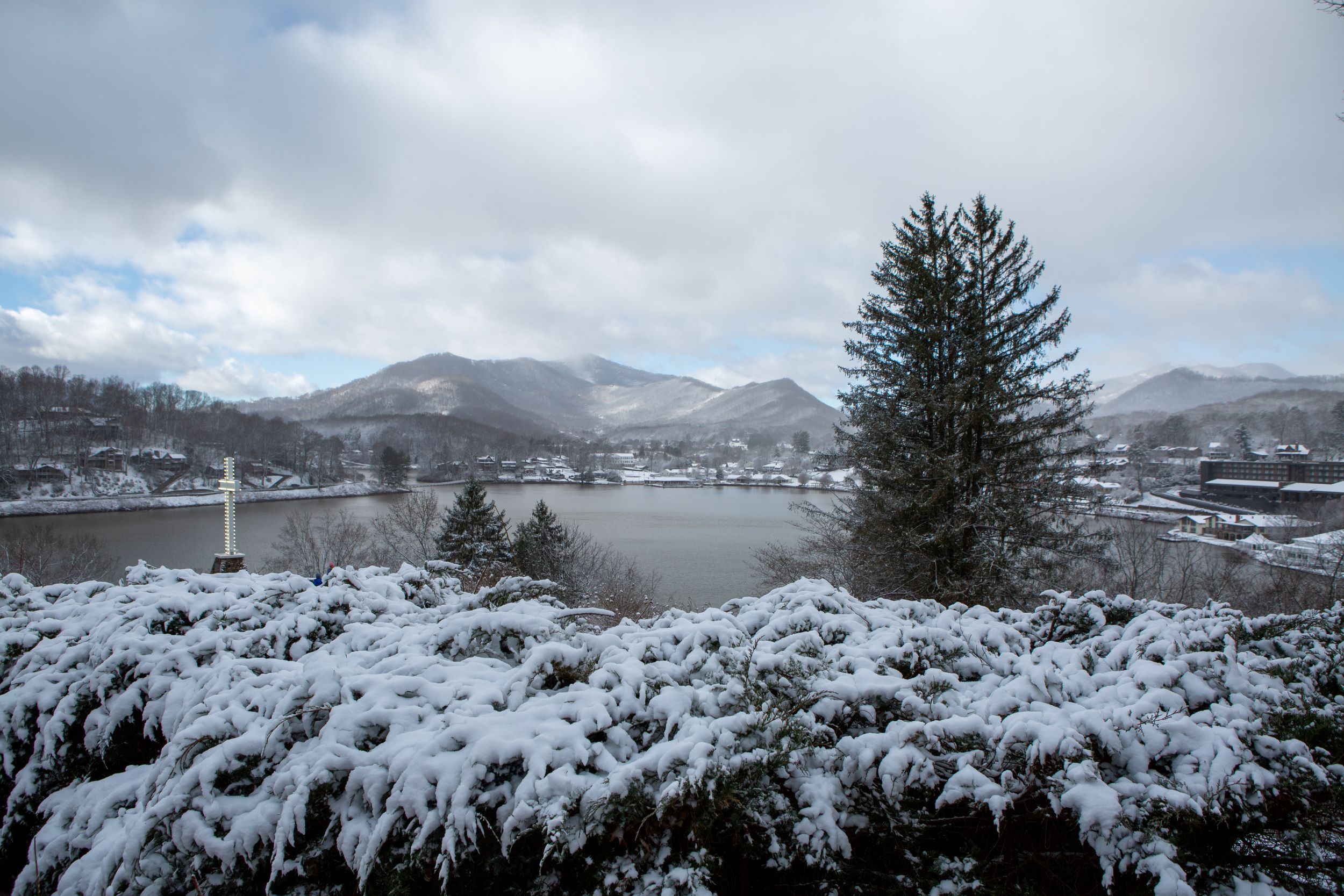The image portrays a wintry landscape of a tranquil lake framed by mountains and dense clouds. The sky, predominantly overcast with gray-white clouds, shows hints of blue peeking through. Charcoal gray mountains form a backdrop encircled by bare trees, leading down to a large, murky gray body of water. To the left foreground, two mid-sized pine trees stand out with their deep green color amidst surrounding dead trees, while a larger pine tree dominates the mid-right, accompanied by snow-covered bushes and pine greenery. Over to the side, a peaceful village is nestled beside the lake, possibly part of a ski resort, adding a cozy, communal feel with suggestions of a house and a white statue near the lake. Snow blankets the entire scene, enhancing the serene, cold ambiance of this black and white image.